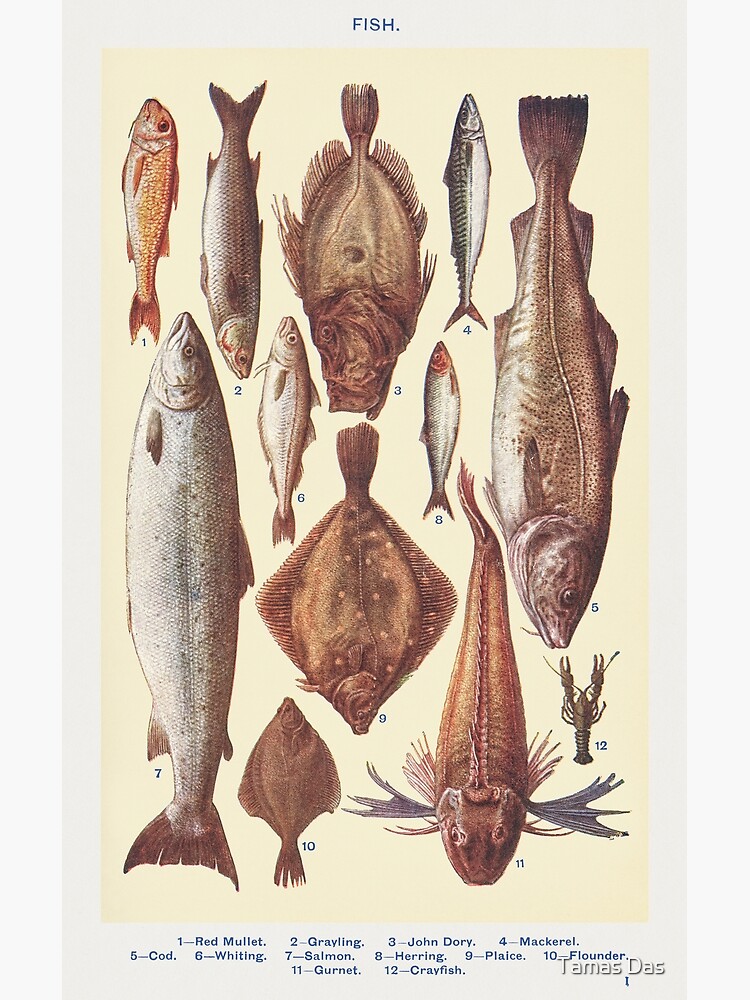The image depicts an intricate, old-timey scientific drawing of 12 different kinds of fish and a crayfish, all meticulously displayed to fit together like a puzzle. Each fish is neatly laid out side by side on a sheet, and they are labeled from number 1 in the top left to number 12 in the bottom right. The names corresponding to the numbers are as follows: 1. Red Mullet, 2. Grayling, 3. John Dory, 4. Mackerel, 5. Cod, 6. Whiting, 7. Salmon, 8. Herring, 9. Plaice, 10. Flounder, 11. Gurnet, and 12. Crawfish. There is also text at the top indicating these are illustrations of fish, and a watermark in the bottom right corner reads "TAMAS DAS."